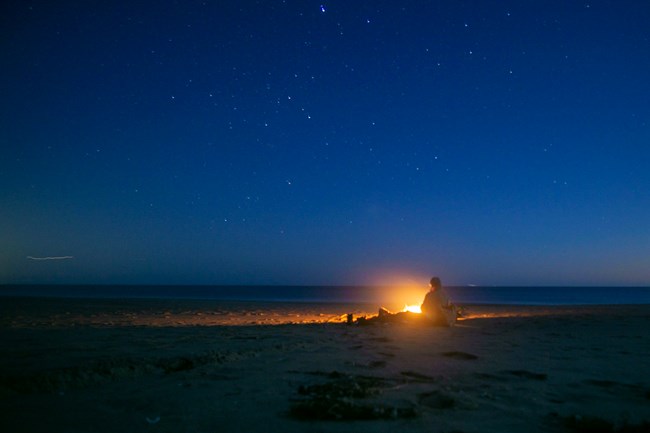In this captivating nighttime photograph of a beach, the serene scene unfolds under a star-studded sky. The upper portion of the image showcases a dark blue that transitions into a lighter blue gradient as it approaches the horizon, reflecting the ocean below. The stars, varying in brightness, sprinkle the heavens, making it a clear and beautiful night.

At the center of the image, a single person sits upright by a glowing bonfire, which casts a bright orange light in all directions, illuminating part of the dark, sandy beach around them. The individual, draped in a blanket and wearing a hat, gazes thoughtfully out over the vast ocean. To their right in the distance, a faint white speck suggests the presence of a distant boat on the water.

The fire’s light and the stars' twinkle create a striking contrast with the dark, tranquil environment, emphasizing the solitude and peacefulness of the setting. The sandy shore appears undisturbed, save for some natural debris like seaweed, adding texture to the foreground. This image beautifully captures the serene essence of a solitary night at the beach, where one can connect deeply with nature and the cosmos.